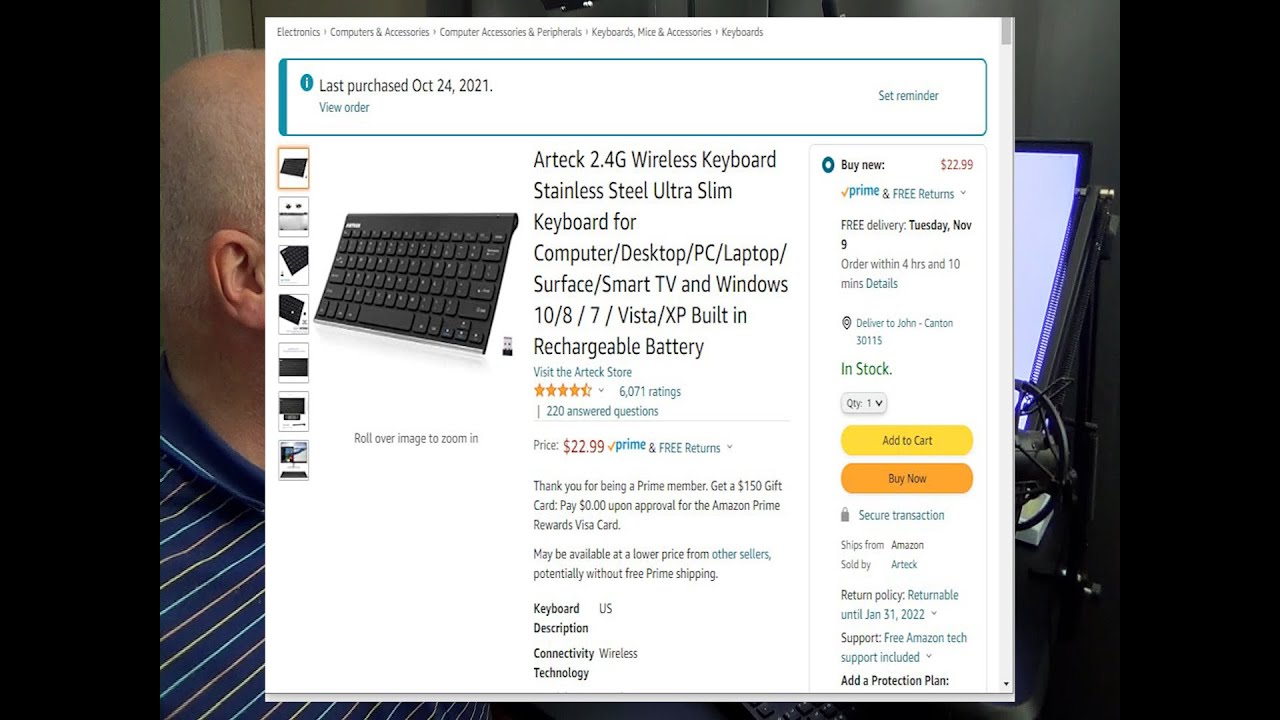**Product Title:** AR Tech 2.4 GHz Wireless Keyboard

**Description:** The AR Tech 2.4 GHz Wireless Keyboard, last purchased on October 24, 2021, is an ultra-slim, stainless steel keyboard designed for use with computers, desktops, PCs, laptops, Surface devices, Smart TVs, and Windows operating systems (compatible with Windows 10, 8, 7, Vista, XP). It features a built-in rechargeable battery and offers seamless wireless connectivity.

**Key Details:**
- **Ratings:** 6,071 customer ratings
- **Questions Answered:** 220
- **Price:** $22.99
- **Shipping Options:** Prime free returns
- **Special Offers:** 
  - $150 Amazon gift card opportunity
  - $0 upon approval for the Amazon Prime Rewards Visa card
  - Potential lower prices from other sellers (may not include Prime shipping)
- **Availability:** In stock 
- **Delivery:** Free delivery by Tuesday, November 9th (order within 4 hours, 10 minutes)
- **Shipping Information:** Ships from Amazon, sold by AR Stock
- **Return Policy:** Returnable until January 31, 2022
- **Support:** Free Amazon tech support included
- **Additional Purchase Options:** Add a protection plan

**Purchase Options:**
- **Add to Cart**
- **Buy Now**
- **Secure Checkout:** Features a padlock for assurance

**Delivery Address:** John Carton, 30115

This highly rated and versatile keyboard is an excellent addition to your tech accessories, promising both style and functionality.